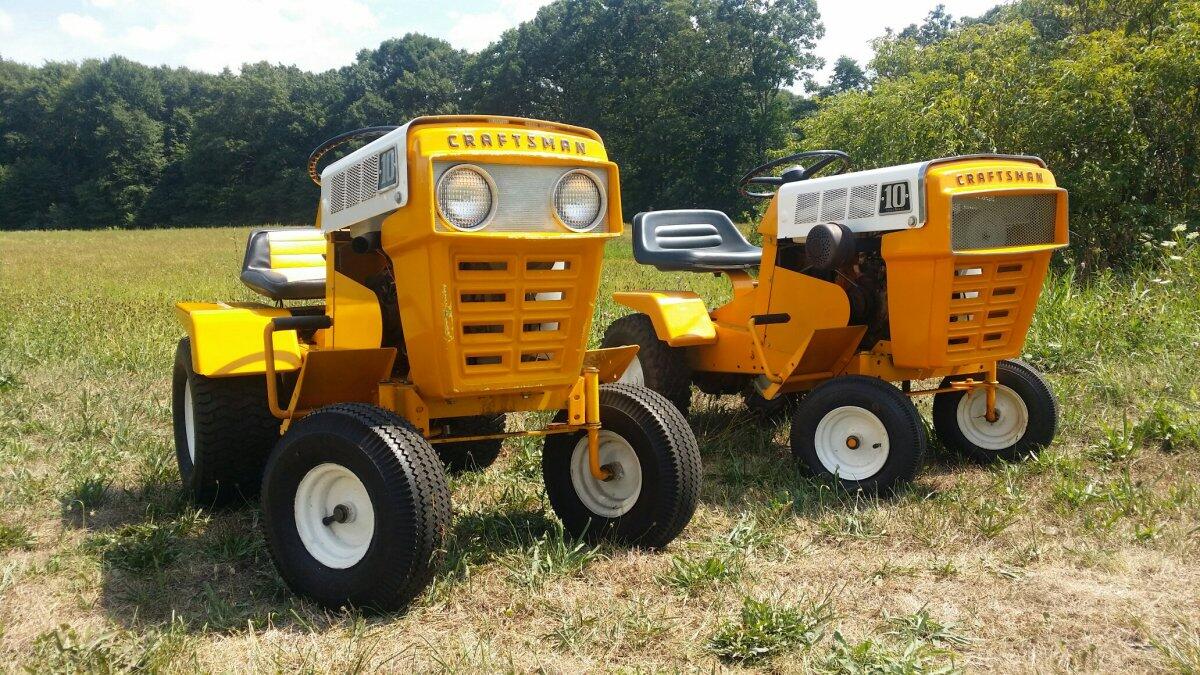The image depicts two small, bright yellow tractors branded by Craftsman, positioned side by side in a grassy field bordered by tall green trees. The tractors, identical in design, feature a prominent yellow front grill with two high-mounted headlights encased in silver brackets. Each tractor is equipped with four chunky black tires with white rims and a black steering wheel. The seating consists of one black plastic seat and one black seat with a large white stripe. The top covers of the engines are white, adorned with the number 10. The tractors lack any covering or roof, with seats exposed like typical farm machinery. They appear designed for light-duty tasks, given their construction and modest tire size. The setting's lush greenery contrasts with patches of dead grass around the tractors, emphasizing their outdoor location and use.